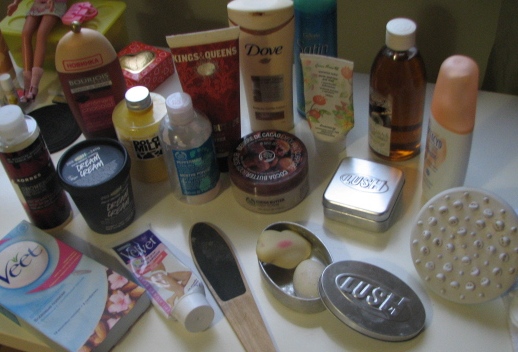A meticulously organized skincare routine is laid out on a pristine countertop. From left to right, the collection includes a bottle of VEET facial cleanser, neatly positioned beside a container of Velvet shaving cream. A nail file rests next to a jar labeled "Lush," presumably filled with fragrant bath salts. 

Parallel to these, a series of products are arranged above: a tub marked "Cream" sits adjacent to a bottle labeled "Milk Lotion." A Dove product, likely a moisturizing cream, completes the display, alongside several other assorted creams. The entire setup showcases an array of skincare essentials, highlighting a comprehensive and well-thought-out self-care regimen.